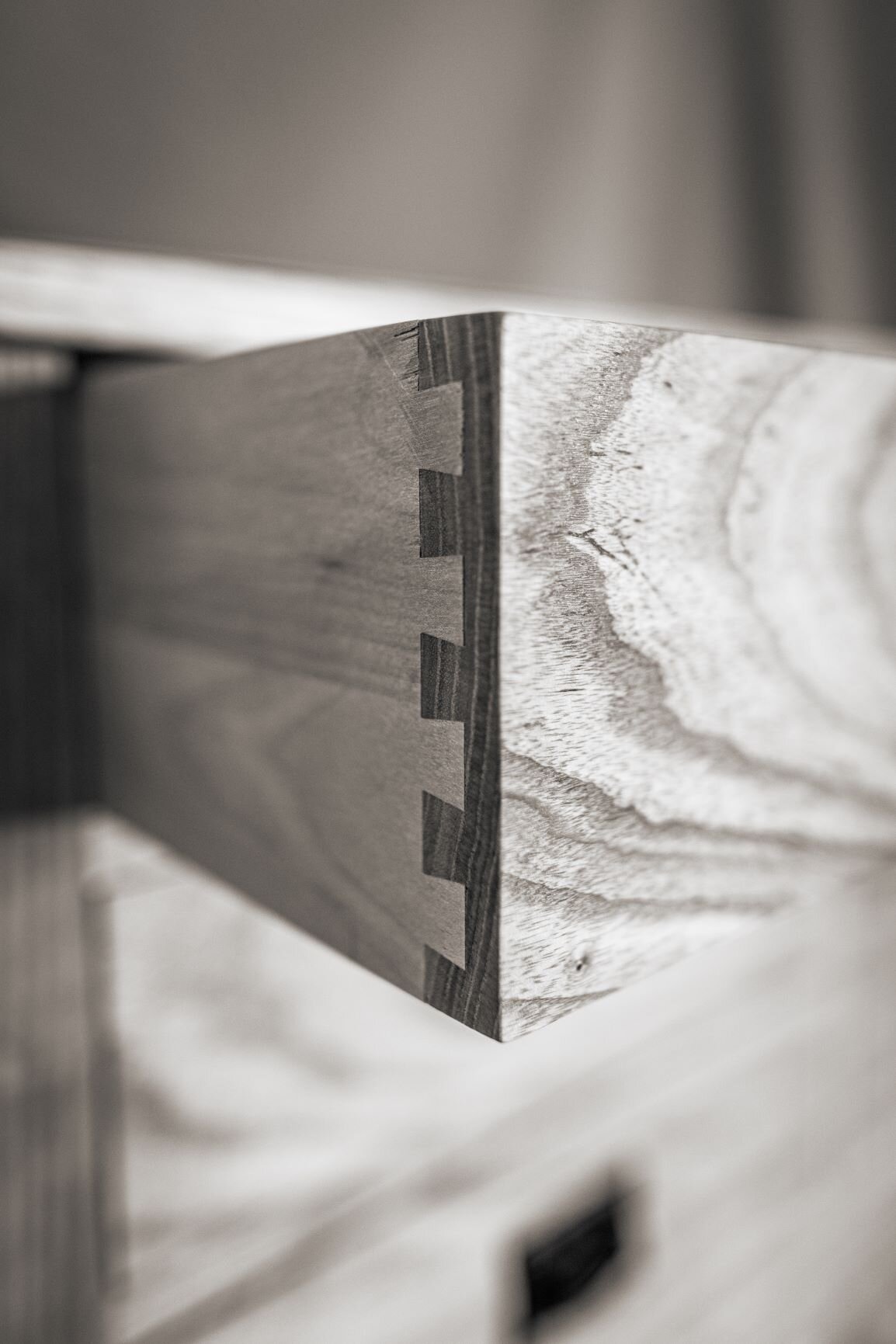The image captures a macro, close-up view of a beautifully crafted, pulled-out drawer made of light gray, weathered wood. The main focus is on the meticulously constructed dovetail joint at the corner, showcasing its tight and well-made fit with dovetail teeth that look almost comb-like, joining the side and face of the drawer seamlessly. The top-most drawer is pulled out, revealing a vertical alignment of at least two more drawers beneath it, though these lower drawers are notably out of focus, contributing to the image's emphasis on the joint. This blurry backdrop trails off with subtle hints of the wood grain and the shape of the handles. The foreground includes an L-shaped metallic object with a wood finish following the contour of the joint, and some indistinct, blurry elements that might be part of a table surface. A shadowed, dark object in the bottom right adds a slight element of mystery, further drawing attention to the intricacy of the dovetail joint. The wood in the image exhibits grain patterns, both on the drawer face and sides, enhancing the tactile richness of the photograph.